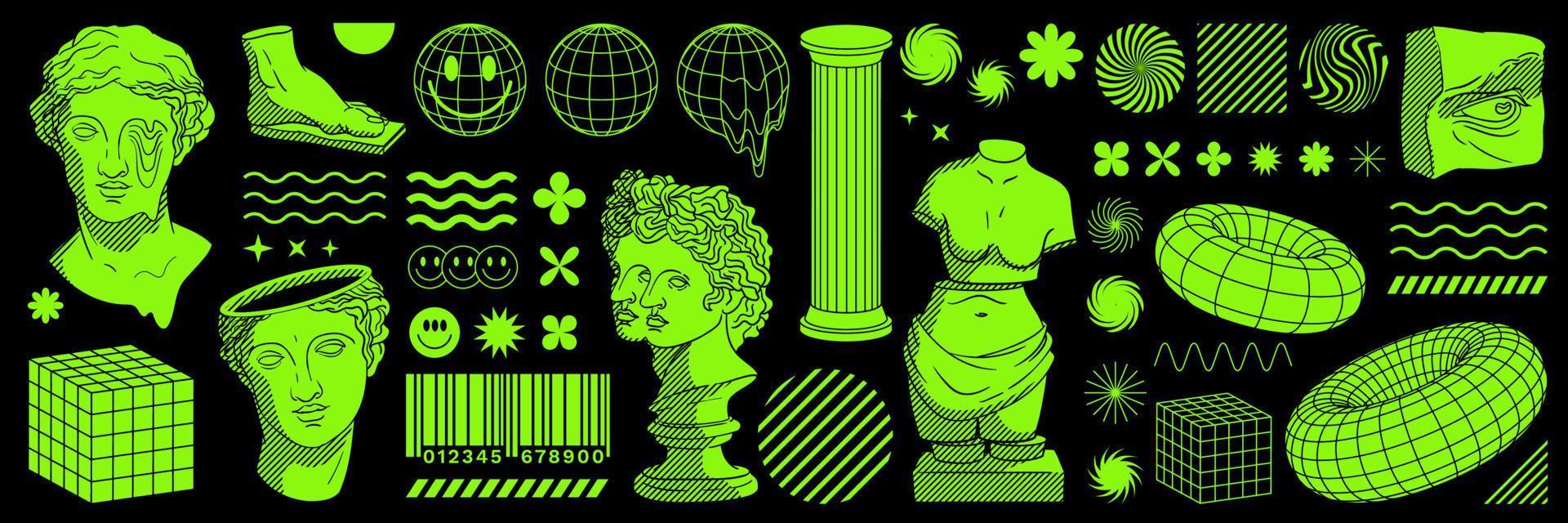This is an intricate horizontal illustration presented on a solid black background, featuring numerous items meticulously drawn in bright neon green. The artwork is a compilation of smaller images, creating a collage-like effect. Predominant among the depictions are elements of classical statuary and geometric shapes. Notable items include various busts of heads, one with the right eye melting, another missing the top part of the skull, and a two-headed sculpture. There are also representations of a disembodied sculpted foot, a nude torso of a woman, and a Greek column. Scattered amongst these are a Rubik's Cube, a barcode, several smiley faces, a melting globe, and other geometric shapes and swirly designs. Each component is evenly spaced across the black canvas, rendered in fluorescent green paint or ink, contributing to the illustration's striking and surreal visual impact.